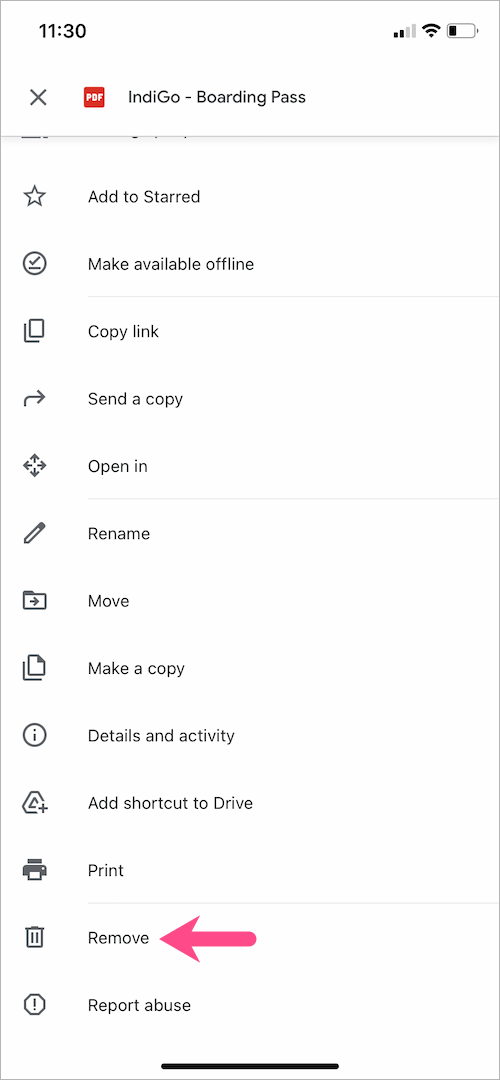The image appears to be a screenshot of a mobile phone interface displaying a list of options for a document or file. At the top of the screen, there is a status bar. In the top left corner, it reads "11:30" in black text. On the right side of the status bar, there are icons for mobile signal strength, Wi-Fi, and battery level, which is nearly depleted.

Beneath the status bar, there's a header area with a white background and predominantly black text. On the left side of this header, there's an "X" icon and a small square possibly reading "ND Go" or indicating a boarding pass. 

The main body of the screen contains a detailed list of options for the document/file, accompanied by black and white icons:

1. Add to star
2. Make available offline
3. Copy link
4. Send a copy
5. Open in
6. Rename
7. Move
8. Make copy
9. Details and activity
10. Add shortcut to Drive
11. Print
12. Remove

Next to the "Remove" option, a dark reddish-pink arrow points towards it. Additionally, a small triangle on the left-hand side points towards the "Remove" option as well.

At the very bottom, there's an option to "Report abuse."

Thin horizontal lines separate some of these options: under the main header logo, under "Make available offline," under "Open in," and under "Print."

There is a black band at the bottom of the screen that spans about halfway across and is centered horizontally.